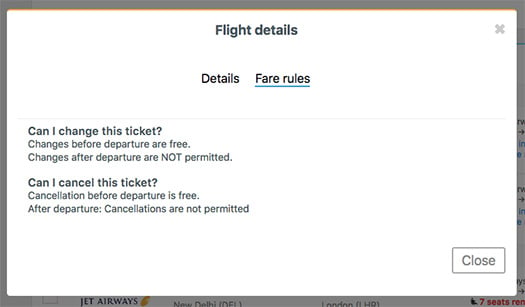The image is a cropped screenshot taken within a flight booking app, layered on top of another webpage or screenshot. It has a clean, white background. Displayed prominently at the top center in dark blue text is "Flight Details," while a grey-colored "X" in the top right-hand corner provides an option to close the window. Directly below "Flight Details," the word "Details" is displayed in black font, followed by "Fare Rules" underlined in blue. 

The screenshot further breaks down into two informative sections. The first section, titled "Can I change this ticket?", states that changes before departure are free, but changes after departure are not permitted. The second section, titled "Can I cancel this ticket?", indicates that cancellations before the departure date are free, whereas cancellations after departure are not permitted. An inconspicuous button to close the tab is located in the bottom right-hand corner. This meticulous layout ensures that users can quickly access essential flight modification and cancellation policies.